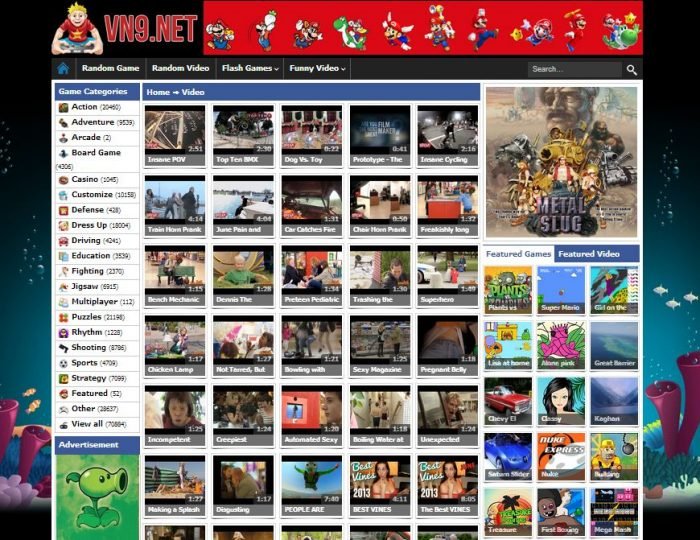The image displays a webpage from vn9.net. Dominating the top of the page is a vibrant red banner adorned with characters from the Mario Brothers franchise, prominently situated towards the center and right. On the left side of this banner, "vn9.net" is emblazoned in very large letters next to a playful cartoon image of a boy holding a remote control. Directly below the banner, the navigation begins with a "Home" button on the left, followed by a row of categories: "Random Game," "Random Video," "Flash Games," and "Funny Video," the last two featuring drop-down menus for additional options. On the far right of this navigation bar, there is a search bar for convenient browsing.

Beneath the navigation bar on the left, a panel starts with a blue header reading "Game Categories." This section lists a vertical menu of various game genres such as Action, Adventure, Arcade, Board Game, Casino, and many more. At the very bottom of this list, a link labeled "View All" displays the total number of available categories, which is 70,884.

The main content area in the center of the page is a vibrant mosaic of video thumbnails, arranged in a grid format. Each row contains five thumbnails, and there are six fully visible rows, making a total of 30 thumbnails on display. These thumbnails likely represent a range of video content available on the site, adding a visually engaging element to the webpage.